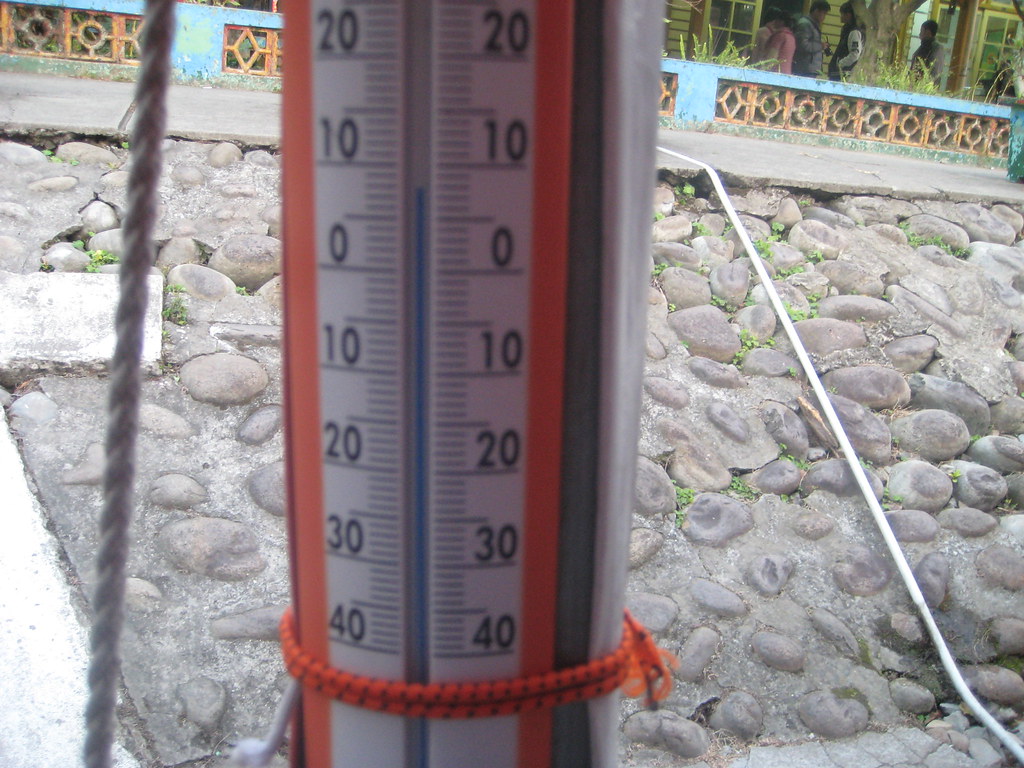In the foreground of this outdoor image, a thermometer is prominently displayed, affixed to a pole with an orange shoelace or rope. The thermometer, which features a white background with black markings, displays temperatures ranging from -40 to 20 degrees Celsius. The blue indicator shows a temperature of 8°C. The thermometer itself is encased in an orange frame. The ground beneath is covered in stones, suggesting this could be part of a backyard setting. A railing is visible in the midground, and an overhead wire extends across the scene. In the distant background, tall grass and several people can be seen near a large tree. Beyond them, windows of a house are partially visible, likely indicating a neighbor's property. The entire scene is bathed in daylight, adding to the clarity and detail of the image.